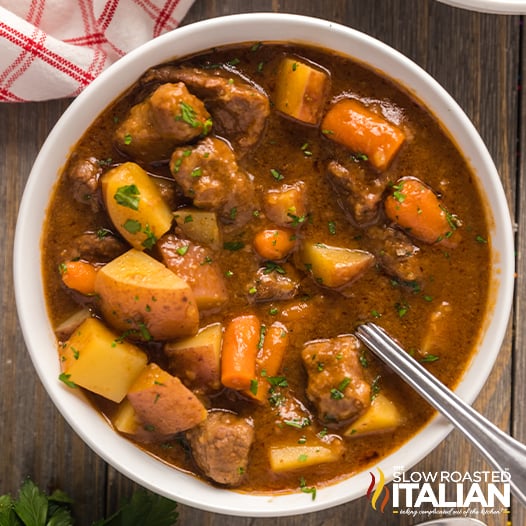This image showcases a hearty bowl of beef stew, perfect for a recipe site. The stew, rich and glistening with a reddish-brown broth, is filled with tender chunks of meat, potatoes, and carrots, garnished with sprinkles of green parsley. The dish is presented in a pristine white bowl, with a silver spoon resting in the stew, ready for tasting. The bowl sits on a dark brown wooden table, adding a rustic touch to the presentation. In the top-left corner of the image, a white napkin with red checkered stripes adds a cozy, homey feel. At the bottom-right corner, the text "Slow Roasted Italian" is prominently displayed in white, accompanied by a small flame icon with shades of red and yellow, indicating a warm and comforting meal. Additionally, leaves of a plant peek from the bottom-left corner, enhancing the natural, fresh theme of the dish.